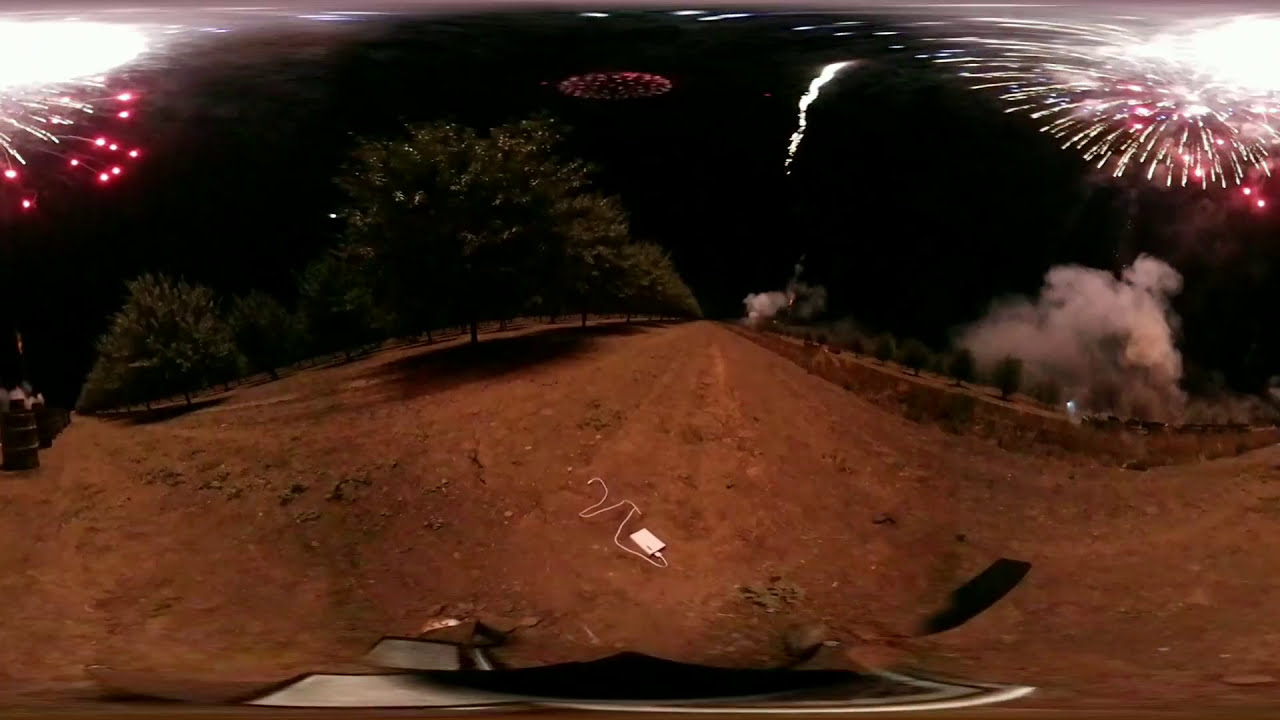This photograph features a distorted, fisheye-lens-like view of an outdoor scene dominated by brown earth, suggesting either a dirt road or an orchard. The nighttime sky is pitch black, providing a stark contrast against the vibrant green trees scattered across the background. Positioned in the upper left, middle, and right sections of the image, red and white fireworks burst dramatically, their sparks lighting up the dark sky and filling it with dynamic energy. Wisps of smoke from the fireworks trail down towards the center and right-hand side of the image, creating a puffy white cloud that stands out against the darkness. In the bottom middle of the picture, a white phone and charger are visible, adding a peculiar modern touch to an otherwise rustic setting. Additionally, a mysterious black and white object at the very bottom of the image remains unidentified, contributing to the enigmatic atmosphere of the scene.